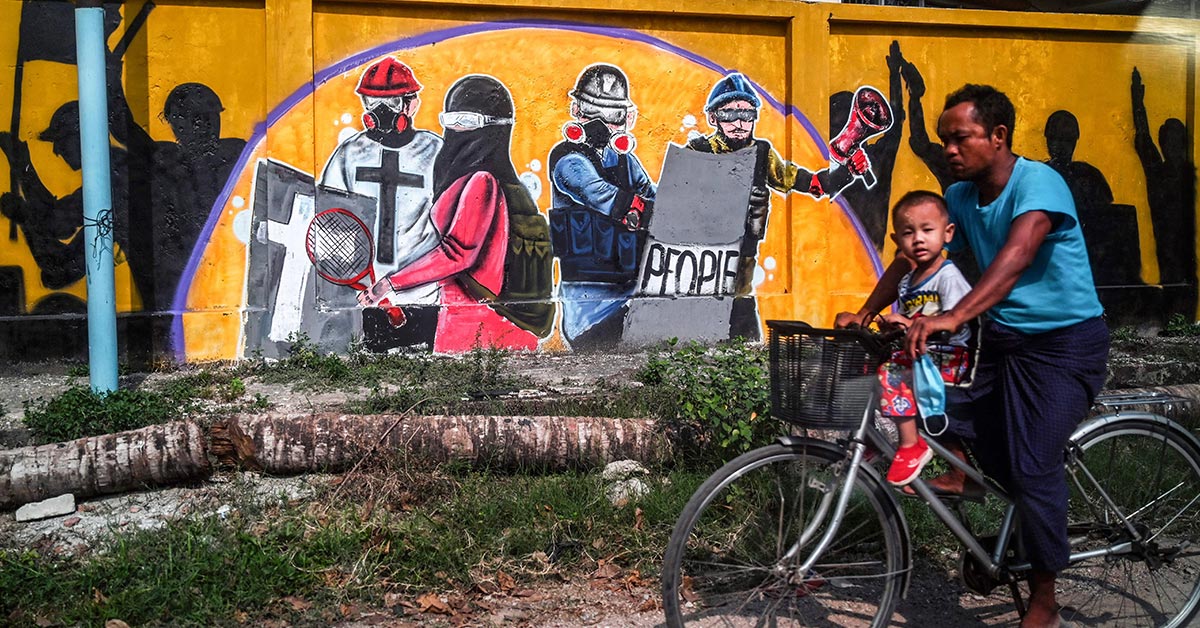The photograph captures a vibrant scene of a darker-skinned man, possibly Filipino, with short black hair, riding a silver bicycle on a clear, sunny day. He is wearing a light blue t-shirt and dark blue baggy sweatpants. Seated in a black basket on the front of the bike, just behind the handlebars, is a little boy, about two years old, dressed in a white shirt, red shorts, and red shoes. They pedal from the left side of the image towards the right, passing alongside a striking mural.

The mural, painted on an orange-yellow wall, teems with evocative graffiti. Dominating the mural is a bluish-purple arch under which four individuals are depicted. To the left, a figure dressed in a red long-sleeve shirt and black ski mask holds a red tennis racket. Nearby, another person wears a firefighter's helmet and a gas mask, sporting a white shirt marked with a black cross. To the right, two figures likely representing law enforcement officers stand with a large gray shield emblazoned with the word "PEOPLE." The mural features additional figures in black, shadow-like silhouettes, stretching across the wall, enhancing the mural's intense and dynamic narrative.